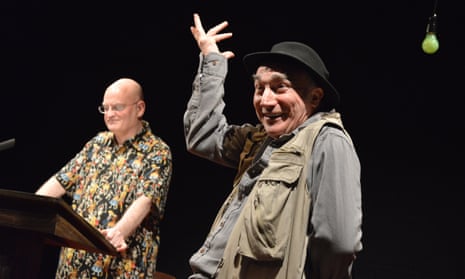The image features a stark black background and highlights two men. The man on the left is bald, wears glasses, and is standing behind a podium adorned with a microphone. He sports a colorful shirt with a black base and vibrant orange, gold, yellow, and small blue patterns. His gaze is fixed on something atop the podium. On the right, another man strikes a dynamic pose with his right arm raised and fingers spread, suggesting a gesture of surprise or emphasis. He wears a black hat, a dark gray long-sleeved shirt, and a khaki vest that gives a rugged, outdoorsy look. He has a broad smile, heavy eyebrows, and notable wrinkles that accentuate his aged appearance. Completing the scene, a green bulb is positioned in the upper right-hand corner, adding an intriguing element to the composition.